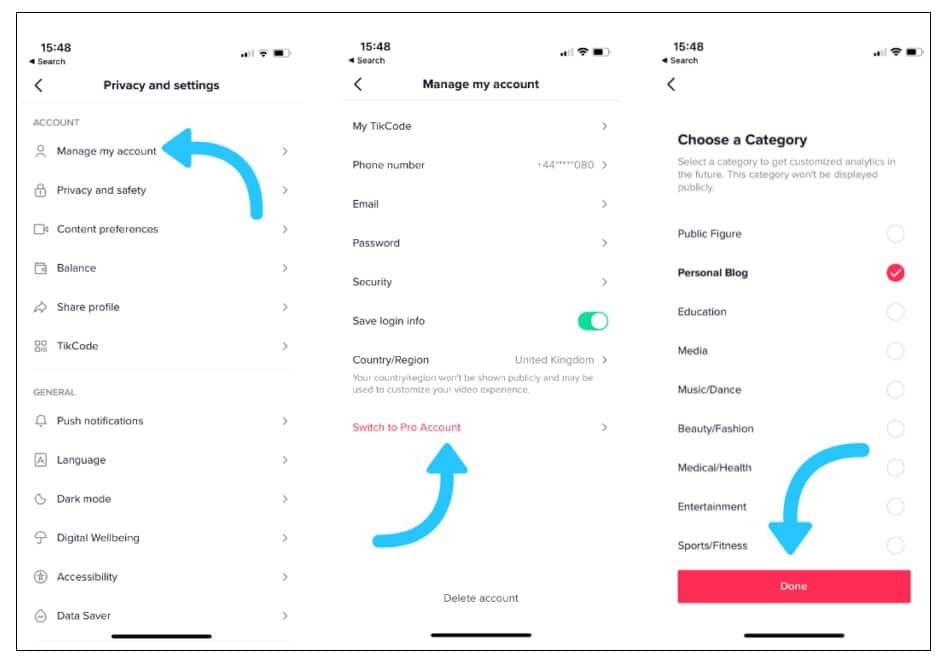This image comprises three phone screenshots captured consecutively, indicated by the uniform timestamp of 3:48 PM (15:48) displayed on the top left of each screenshot, and a consistent battery life of approximately 70% shown at the top right.

The first screenshot on the left highlights the "Privacy and Settings" menu. Within this menu, a blue curved arrow directs attention towards the "Manage My Account" option. The menu also features tabs like "General," which includes sub-options such as push notifications, languages, and dark mode. Above it, the "Account" tab lists options including manage my account, privacy and safety, and balance.

The middle screenshot shows the "Manage My Account" screen, which is the next step after selecting the aforementioned option. This screen displays account details such as My TikCode, phone number, and email. At the bottom, another blue arrow points towards an option labeled "Switch to Pro Account" (previously misinterpreted as 'pedo account').

The final screenshot on the right features the "Choose a Category" screen that appears after opting to switch to a Pro Account. This screen lists several categories like public figure, education, and personal blog. The chosen category, personal blog, is highlighted, and a blue arrow points towards the red "Done" button at the bottom of the screen.

Together, these screenshots document the step-by-step process of navigating through account settings to switch to a Pro Account, culminating in the selection of an account category.